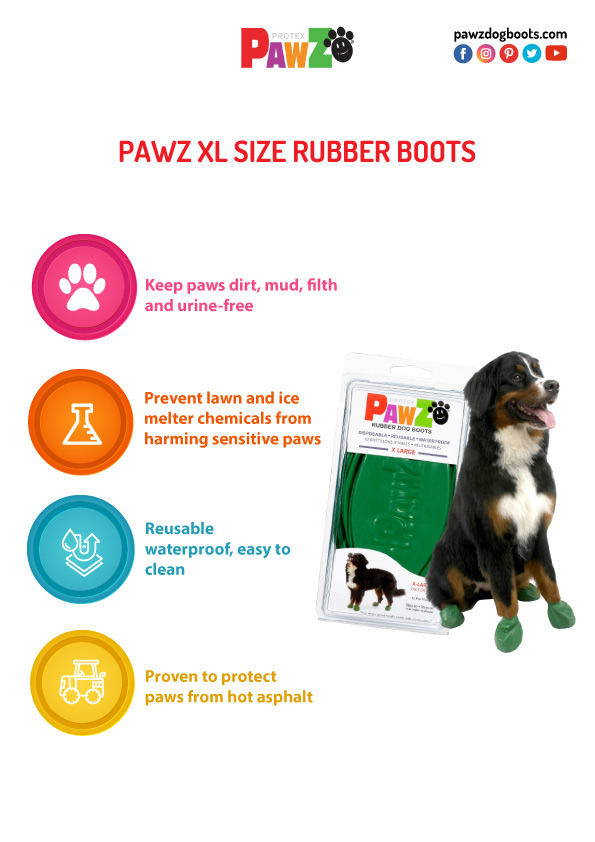The advertisement showcases Paws XL size rubber boots for dogs on a white background. At the top center, "PAWZ" is spelled out in colorful, capitalized letters with a black paw print stamp, and to the right, the website "PawsDogBoots.com" is displayed. Below the website, logos for Facebook, Instagram, Pinterest, Twitter, and YouTube are neatly aligned. In bold red text, the title reads "PAWS XL SIZE RUBBER BOOTS."

Four informational icons are listed in circles below the title:
1. A pink circle with a paw print states, "Keep paws dirt, mud, filth, and urine free."
2. An orange circle featuring a chemistry tube warns, "Prevent lawn and ice melter chemicals from harming sensitive paws."
3. A blue circle with a water droplet indicates, "Reusable, waterproof, easy to clean."
4. A yellow circle with a construction vehicle symbol declares, "Proven to protect paws from hot asphalts."

To the right of these details, the product's packaging is depicted, showing green rubber boots neatly arranged in a bag. Beside the packaging, a medium-sized dog with black, brown, and white fur is wearing the green rubber boots on all four paws, highlighting the practical use of the product.